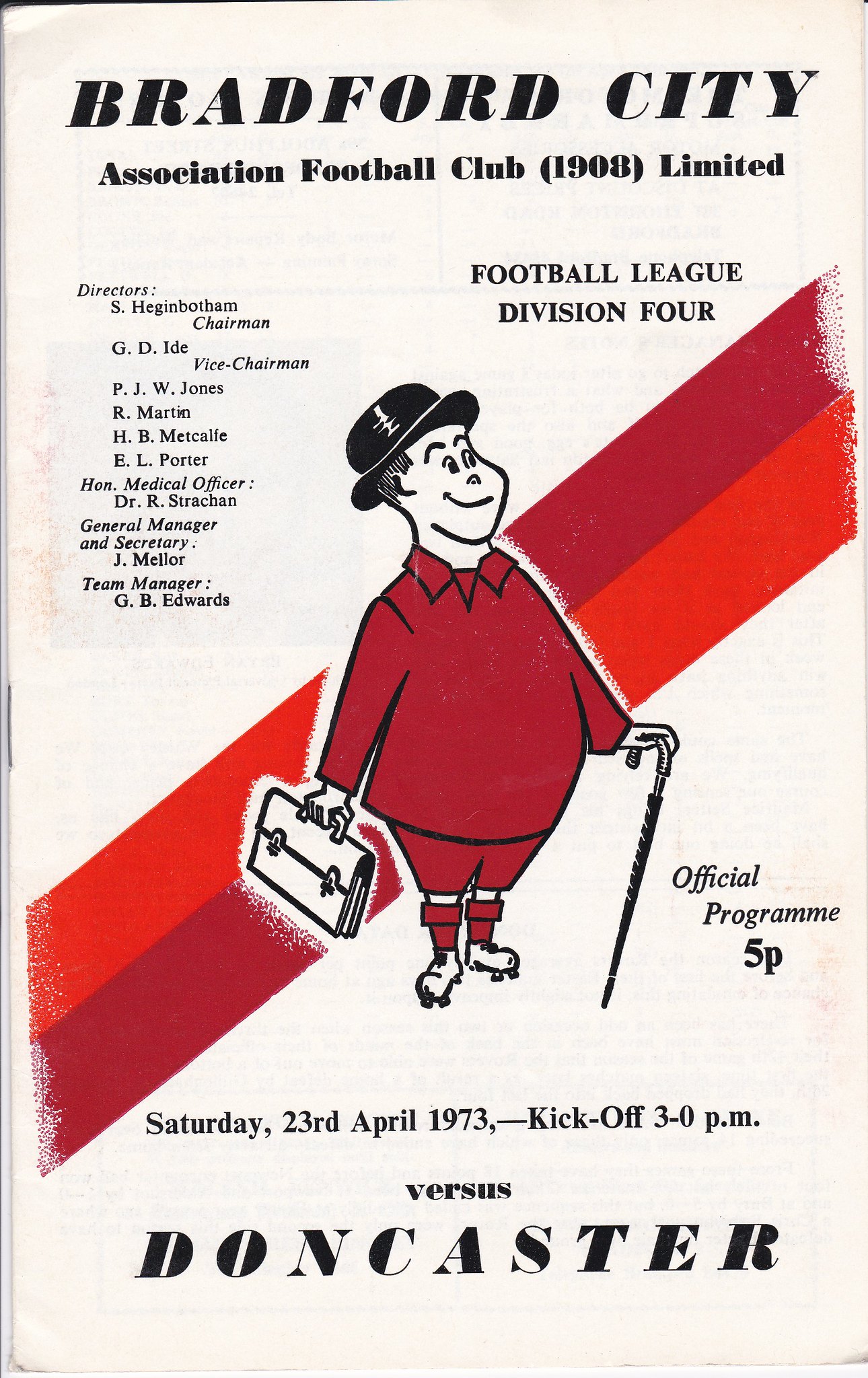The cover of this soccer game day program, which is black and white, features an illustration of a man in the center dressed in a red soccer outfit, including a long-sleeved collared shirt, shorts, knee-high socks, and cleats. He wears a small black top hat and holds a cane or umbrella in one hand and a briefcase in the other. Behind him, two diagonal stripes in shades of red and orange run from the bottom left to the top right, reflecting the team colors. At the top, the text reads "Bradford City Association Football Club 1908 Limited," and "Football League Division IV" follows on the right. There is a detailed list of directors, medical officer, general manager, and team manager on the left. Additional smaller text near the bottom mentions "Official Program, Five Pence, Saturday, the 23rd of April, 1973, Kickoff, 3 p.m., versus Doncaster."